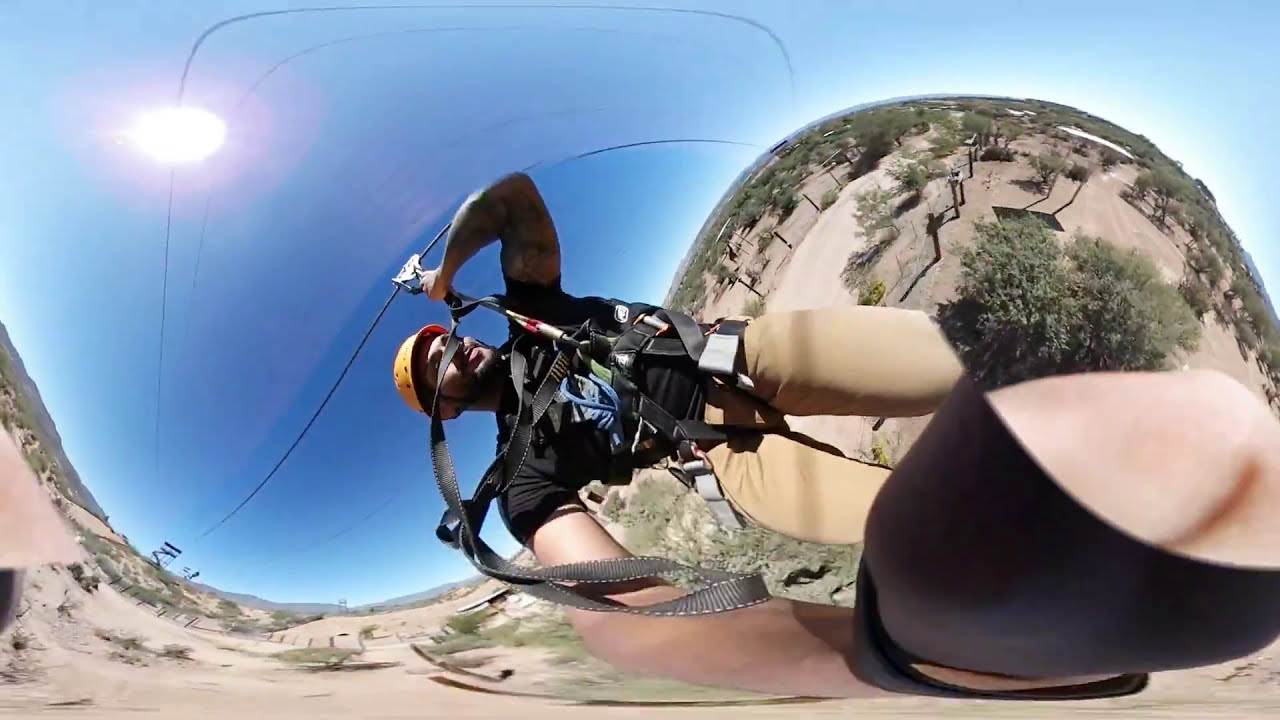The photograph captures a surreal outdoor scene with an unusual distortion effect that creates a wavy, almost fluid appearance. Set in a sandy, flat terrain sparsely dotted with green vegetation under a clear blue sky, the sun shines brightly in the upper left corner. Dominating the image is a young man, around 30 years old, wearing a yellow crash helmet, a black t-shirt, and khaki pants. He is strapped into a black harness, suggesting he's either rock climbing or ziplining. The man’s position is disoriented by the photo's angle; he appears sideways, rotated 90 degrees counterclockwise, as if his head points at nine o'clock. His left hand grips part of the harness, while his right hand extends outward, holding what looks like a GoPro camera, possibly capturing the moment himself. The background further adds to the photograph's peculiarity, with swirling elements that make the terrain and vegetation appear as layers superimposed upon each other, contributing to the sense of a multidimensional, almost dreamlike landscape.